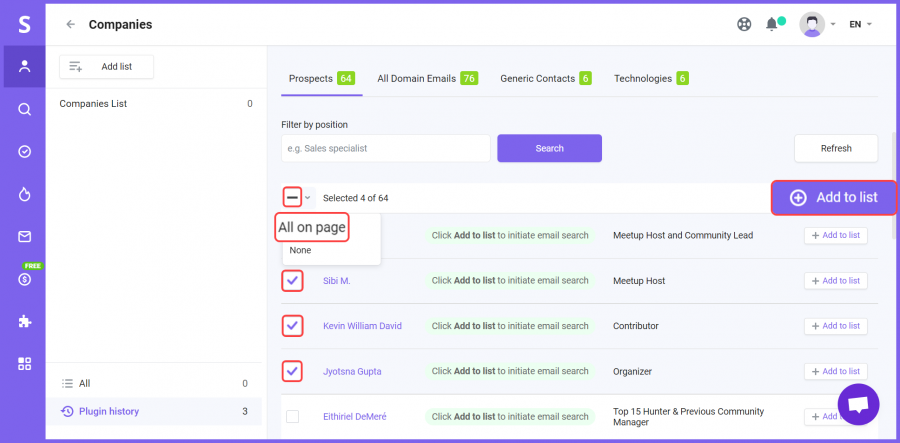In this image, we see a screenshot framed with a purple outline. The left side features a vertical purple bar populated with numerous icons. Adjacent to the purple bar, bold text reads "Companies." In the upper right corner, there is a cartoon-like avatar representing the user, accompanied by a notifications bell and a pull-down menu labeled with the letters "EN." There are multiple links displayed at the top in dark blue text, including "Prospects" which is highlighted with a green box displaying the number 64. Other sections include "All Domain Emails" in a green box with the number 76, "Generic Contacts" in another green box indicating the number 6, and "Technologies" also within a green box showing the number 6.

Below these sections, there is a white form box labeled "Filter by Position" with the placeholder text "e.g., Sales Specialist." To the right of this input box, a blue action button is labeled "Search," and next to it, there is a white button with the word "Refresh."